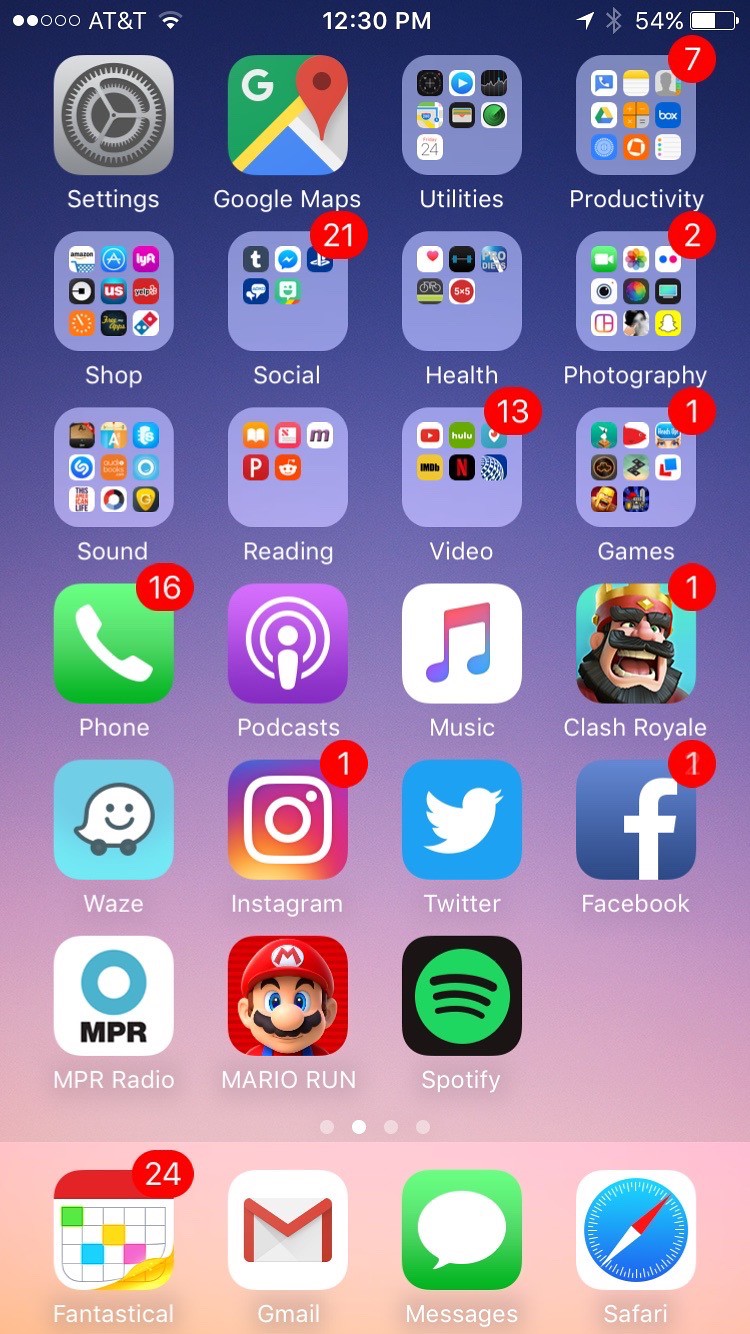This is an image of a smartphone homepage featuring a variety of widgets, many of which display red notification circles with numbers inside them. On the bottom row, the apps include Safari, Messages, Gmail, and Fantastical, which has 24 notifications. The row above features Spotify, Mario Run, and NPR Radio. Further up, prominent apps include Facebook with one notification, Twitter, Instagram with one notification, Waze, Clash Royale with one notification, Music, and Podcasts. The Phone app shows 16 notifications. Adjacent to these, there is a folder labeled "Games" with one notification and another folder called "Videos" with 13 notifications. Additional folders such as "Reading," "Sound," "Shop," and "Social" group several widgets together; the "Social" folder displays 21 notifications. Other notable apps include Health, Photography with two notifications, Productivity with seven, Utilities, Google Maps, and Settings. The status bar at the top-left corner indicates the device is connected to AT&T, with the time displayed as 12:30 p.m. On the right side of the status bar, the battery life is shown at 54%.